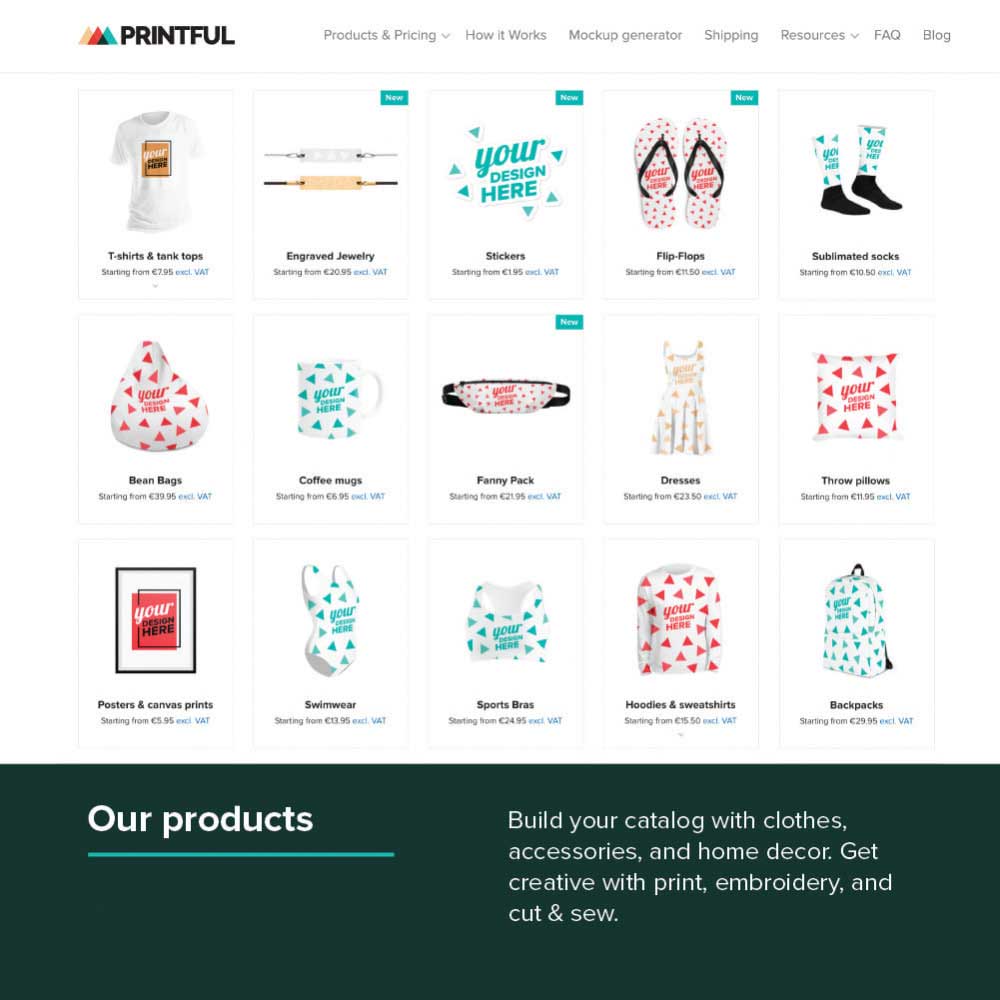This image is a detailed screenshot from the Printful website, showcasing its diverse product range and navigation options. At the top of the screenshot, a navigation bar features clickable links including "Products & Pricing," "How It Works," "Mock-up Generator," "Shipping," "Resources," "FAQ," and "Blog." Below this, the main section is organized into a 5 by 3 grid displaying different product categories. Each category is represented by a square showcasing sample images.

In the first row, the products listed are T-shirts and tank tops, engraved jewelry, stickers, flip-flops, and sublimated socks. The second row features beanbags, coffee mugs, fanny packs, dresses, and throw pillows. The third row includes posters and canvas prints, swimwear, sports bras, hoodies and sweatshirts, and backpacks.

Beneath the grid, a prominent black rectangle with white text underlined in green states "Our Products." To the right, additional text encourages users to "build your catalogue with clothes, accessories, and home decor," inviting them to "get creative with print, embroidery, and cut & sew." Each product category within the grid is accompanied by images illustrating potential design placements for customization.